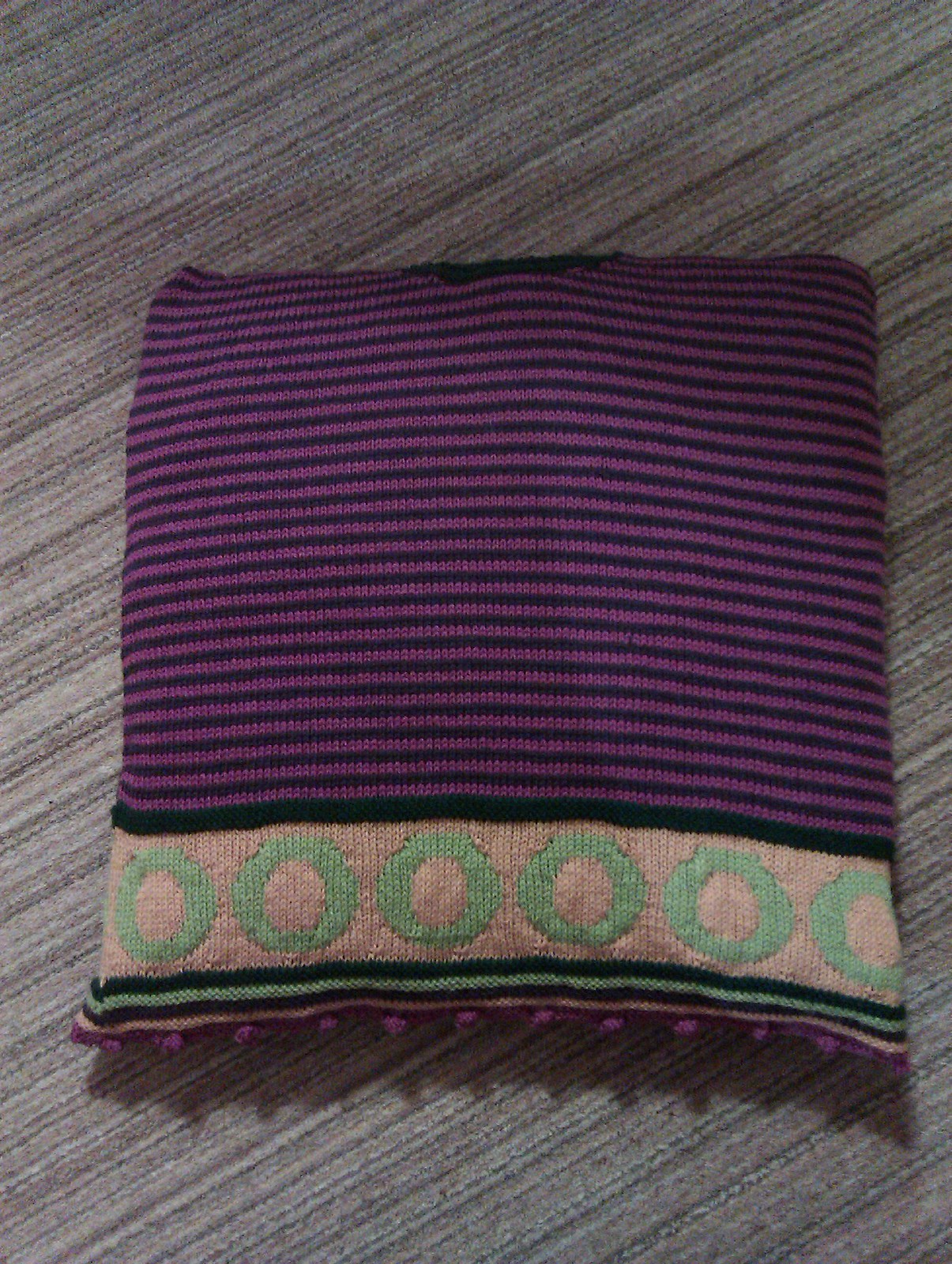This image depicts a vertically aligned rectangular photograph of a decorative throw pillow situated on a striped, gray carpet or rug. The carpet features a thin, blended pattern of darker and lighter gray stripes. The pillow itself is square-shaped and prominently positioned in the center of the image. Its main section, which comprises about four-fifths of the pillow's height, boasts alternating horizontal stripes of purple and black, each of equal width. 

Near the bottom of the pillow, there is a bordered area with a different design. This section is tan and adorned with six large, light green circles embroidered in a row from left to right. Below this tan segment, the pillow displays alternating stripes of black and green, followed by another tan stripe. The very bottom features a final purple stripe adorned with short, tiny purple tassels hanging downward. The intricate design and the setting on the striped carpet create a visually captivating composition.